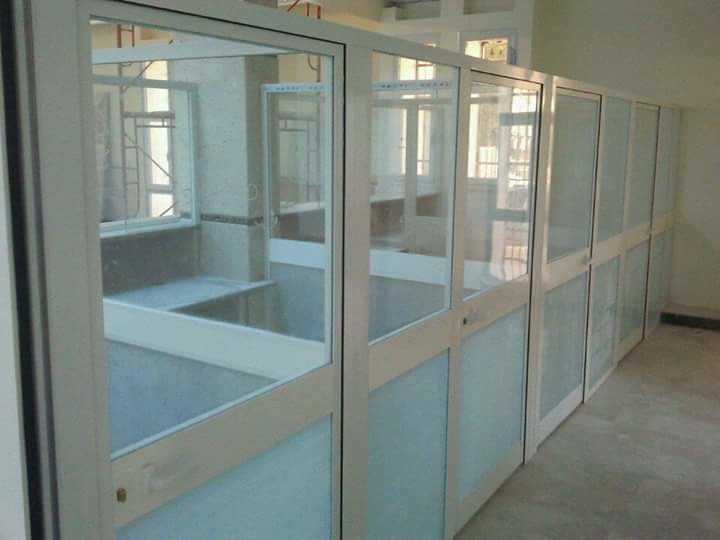This photograph captures the interior of a building under construction, possibly being converted into a bank or another type of secure facility. The scene prominently features a set of three automatic doors with white frames, placed adjacent to each other. Beyond these doors, turning to the right, there appears to be another set of doors leading to a corridor. The space above the doors aligns with their height, forming a linear division within the lobby area.

In the foreground, there are several booth-like structures being assembled, each fitted with a table and a glass viewing area, resembling teller windows or visitation booths. These booths are made with clear materials—likely glass or plastic—enclosed in aluminum frames at the top and bottom. The repetitive design suggests a functional arrangement for privacy and communication, possibly hinting at a bank's customer service area or a prison’s visitation setup.

Moreover, there is scaffolding by large windows on the far side, indicating ongoing construction work. Natural daylight streams through these windows, illuminating the white walls and the cement floor. Overall, the space is an amalgamation of unfinished construction, with scaffolding and booth installations highlighting the transitionary state of this interior.